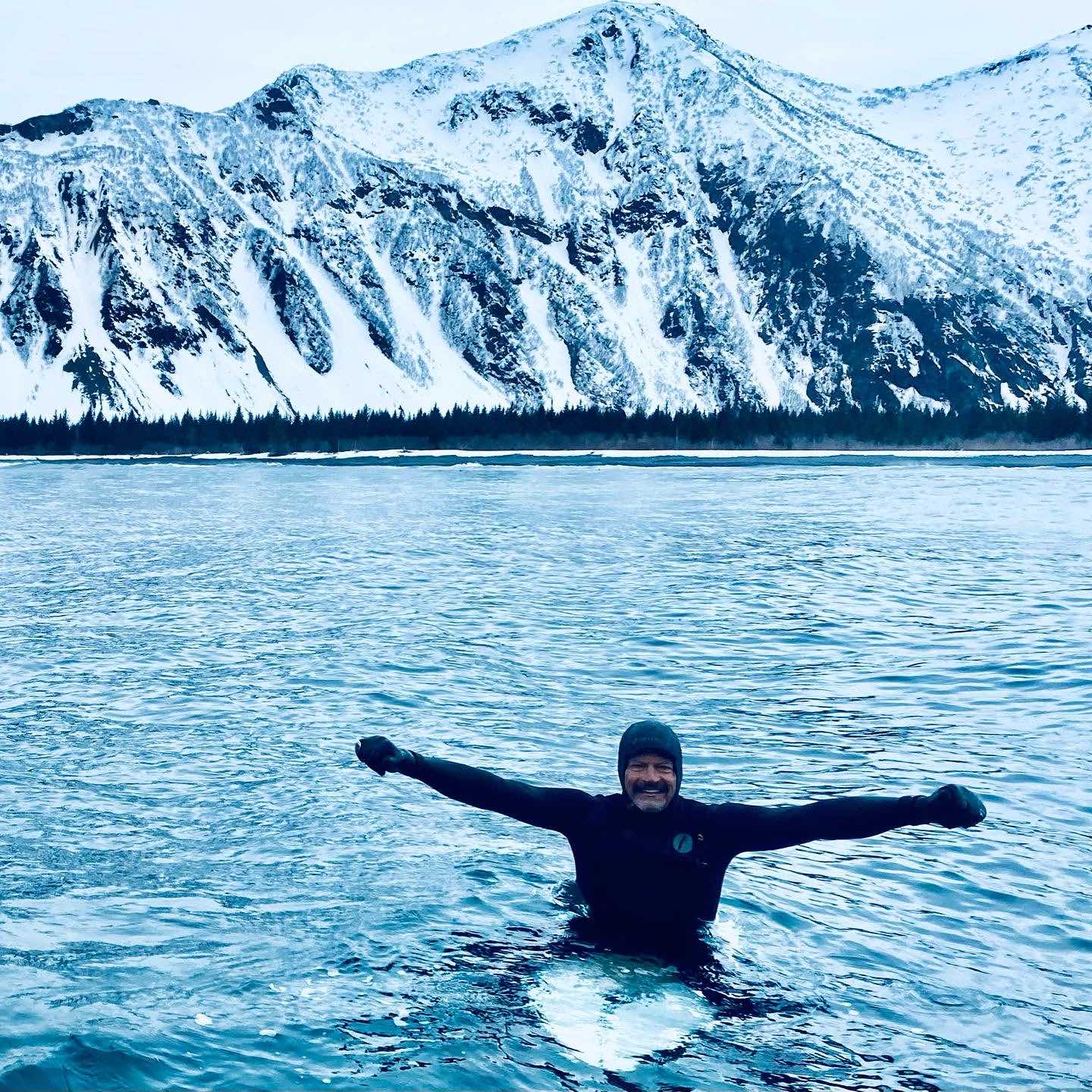In this captivating square-shaped image, a smiling older white man, possibly in his 50s, is seen waist-deep in the icy blue water of a frozen sea or lake. The man, sporting a mustache and beard, is clad in a black wetsuit with a hood, and his gloved fists are extended outward to either side. Behind him stretches a stunning winter landscape, where expansive forested areas give way to a snow-blanketed shoreline. Towering majestic mountains, fully covered in snow rather than just capped, dominate the background, accentuating the frigid, serene beauty of the scene. The man appears to be seated on a partially submerged surfboard, enjoying his time despite the evident cold, illustrated by the pristine, snowy surroundings.